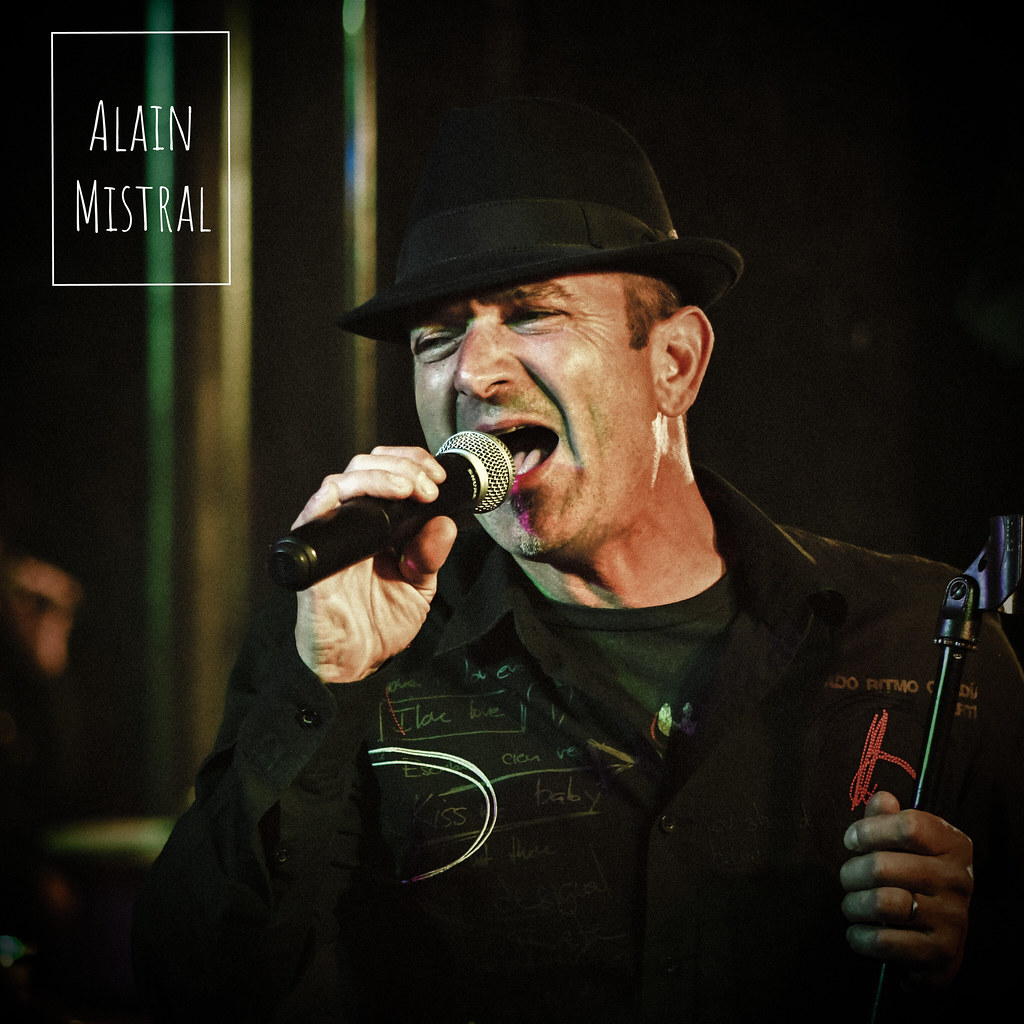In this striking, high-quality image, a middle-aged Caucasian man is captured mid-song, gripping a microphone with a black stem and silver front close to his mouth. His left hand firmly holds a microphone stand, showcasing a wedding ring. He is dressed in a black, long-sleeved collared shirt adorned with writing and logos, with a graphic t-shirt underneath. A black hat with a short brim and a ribbon, tilted forward, complements his thin brown hair and neatly groomed face with a subtle soul patch. The backdrop is a deep, unobtrusive black, with goldish posts faintly visible on either side. The man is slightly off-center towards the right of the frame, and in the top-left corner, the name "Alain Mistral" is prominently displayed in white letters within a white rectangular box.